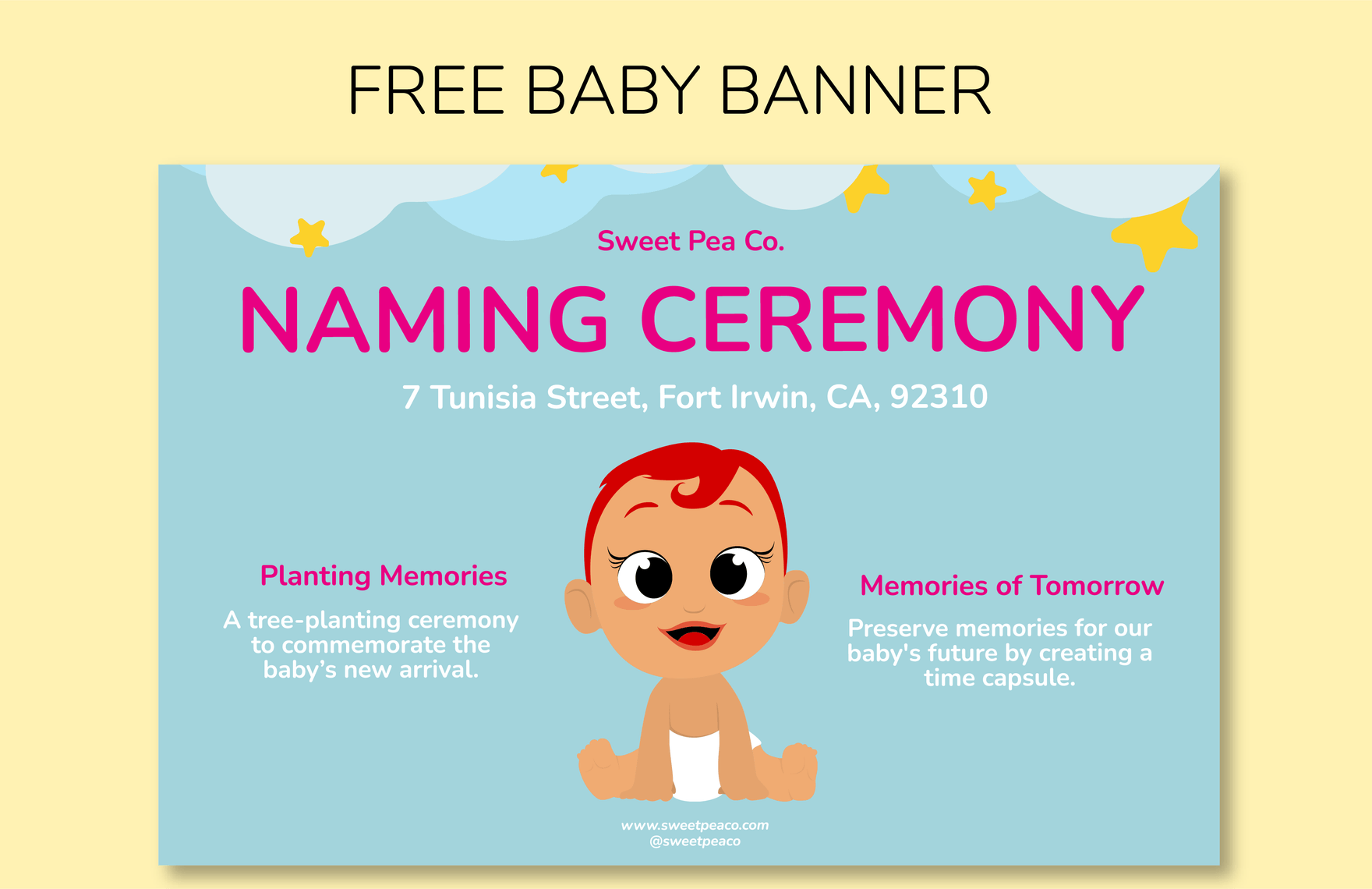This vibrant image showcases a celebratory flyer against a pale yellow backdrop. At the top of the image, bold text reads "FREE BABY BANNER." The centerpiece of this flyer is titled "Sweet Pico Naming Ceremony," set against a soft blue background adorned with whimsical clouds and sparkling stars.

Below the title, essential event details are provided, including the address “7 Tunzea Street, Fort Irwin, California, 92310.” A charming cartoon baby with big, expressive eyes and red hair, dressed in a simple diaper, is prominently featured in the center, adding a playful touch to the flyer.

To the left of the baby, the text "Planting Memories" highlights a tree planting ceremony meant to celebrate the baby's arrival. To the right, "Memories of Tomorrow" invites participants to create a time capsule, ensuring cherished memories are preserved for the future.

Overall, the flyer radiates a sense of joy and anticipation for the special events surrounding the baby's naming ceremony.